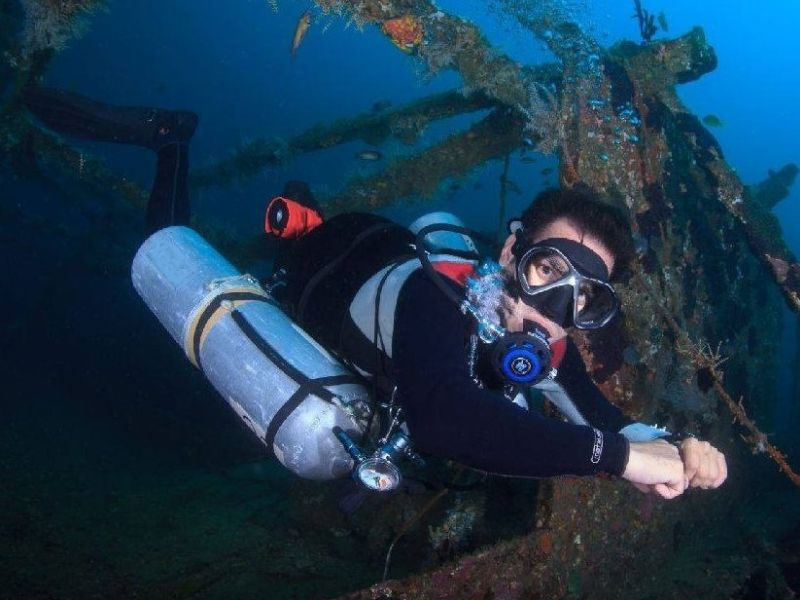This underwater photograph captures the serene yet mysterious scene of a scuba diver exploring what appears to be a submerged wreckage. The water transitions from a lighter blue on the right to a darker, deeper hue on the left, creating an ethereal gradient. In the lower right corner, a man in full scuba gear — including a dark-colored wetsuit with grey accents, large flippers, and a blue oxygen tank — stares directly at the camera through his goggles. His equipment includes a respirator with black tubes attached to the tank, mounted on the side of his torso. His hands are extended in front of him, fists together, with a tiny blue fish adorning his palm. The diver, with his brown hair visible under his equipment, appears to be navigating through a rusted shipwreck, where diffuse, cobbled wooden pieces encrusted with undersea growth can be discerned in the background. Although other small fishes are barely visible, they add a touch of life to the otherwise somber scene.